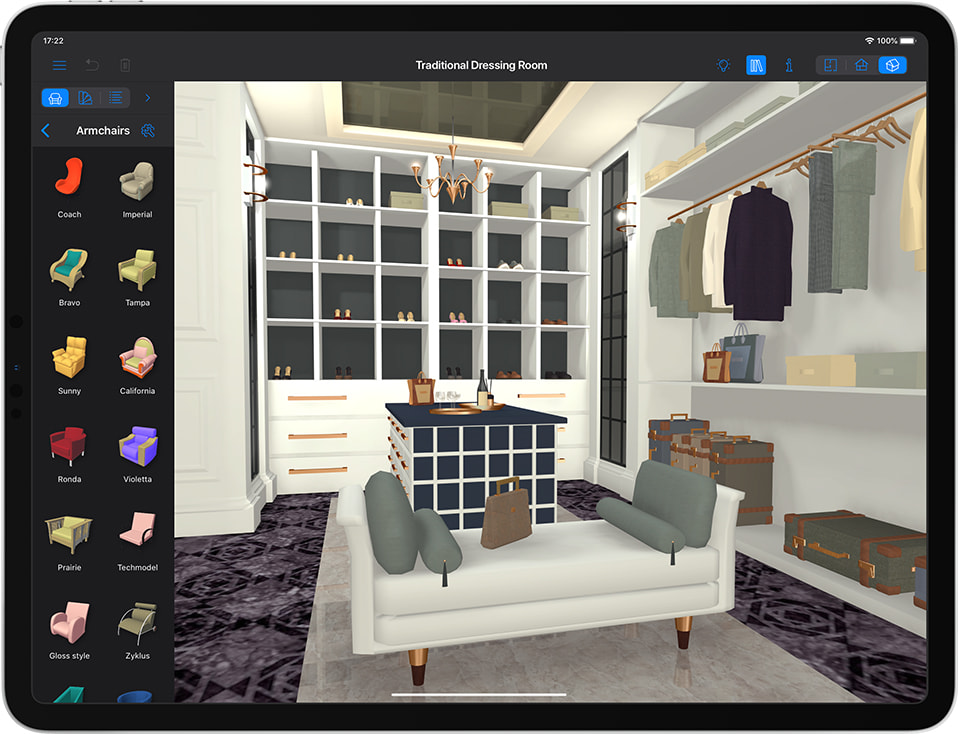This image is a detailed, computer-generated depiction of an opulent and spacious dressing room or closet, designed within an interior design application. At the back of the room, there is a built-in wall featuring cubicle shelves filled with an array of digitally rendered shoes, and beneath these shelves, a set of six drawers. Centered in the room is an island with multiple drawers, adorned with glasses and plates on its black tabletop. In front of the island is a plush white ottoman-like sofa, which holds a handbag and four gray pillows.

To the right, a rack offers ample space for hanging clothing, with additional shelves below for storing purses and boxes, and space on the floor for luggage and travel trunks. The room's aesthetic is underscored by a decorative chandelier hanging from the ceiling. The color scheme includes gray flooring, a blue and white island, and gray and blue suitcases, while the drawers and shelving are uniformly white and gray. The left side of the image displays a selection of armchairs in various styles and colors, highlighting the customization features of the design application.